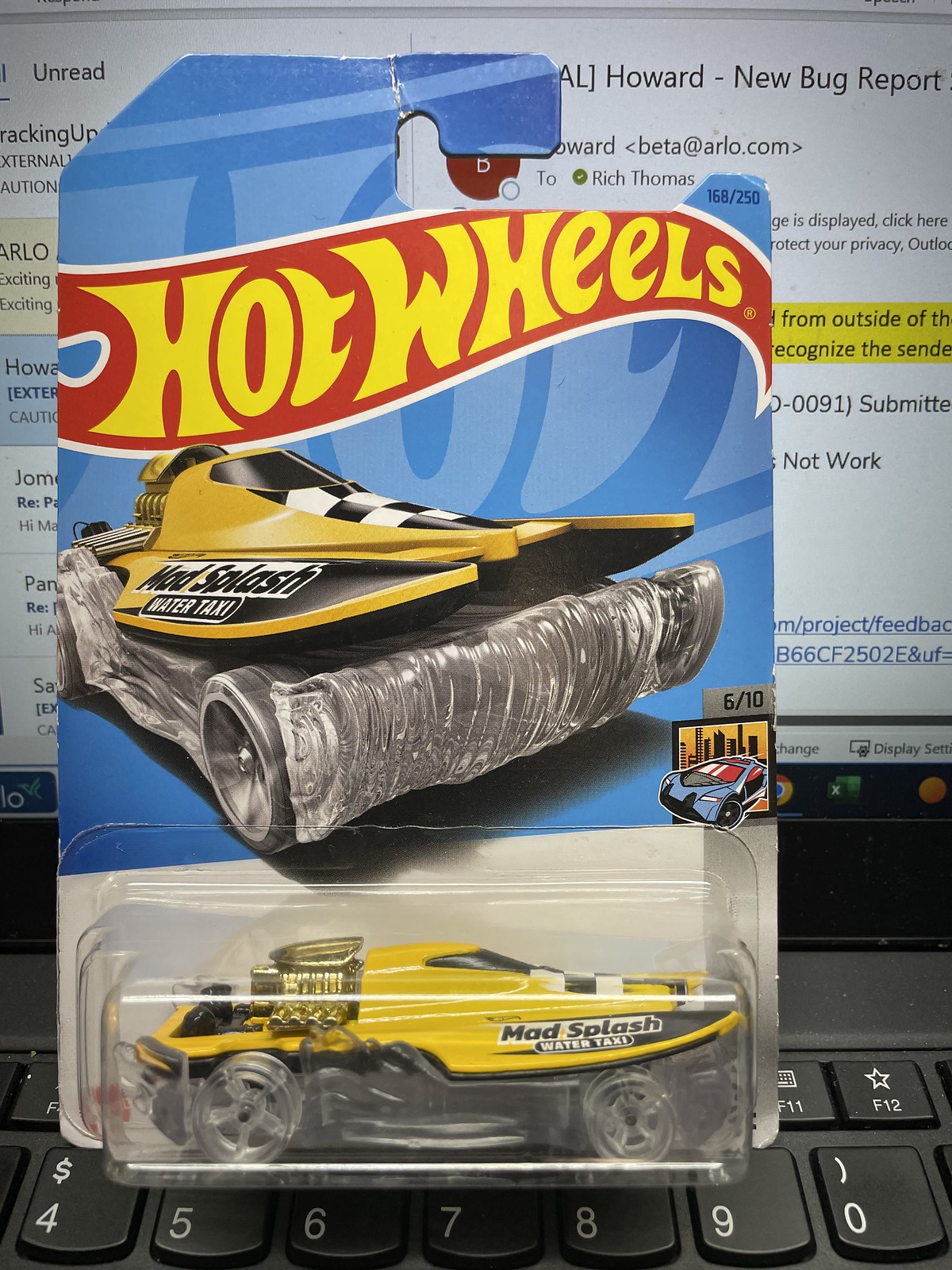The image depicts a detailed scene centered around a Hot Wheels car still in its original packaging. The car, a yellow "Mad Splash Water Taxi" with a distinctive shape resembling a jet ski, features a prominent gold engine mounted at the back, clear white wheels, and a black undercarriage. The toy is encased in classic Hot Wheels packaging, characterized by a blue background and the iconic red banner with yellow block lettering reading "Hot Wheels" at the top. Positioned in the foreground, the package is standing upright on a black laptop keyboard. The laptop is powered on, and the screen displays a document titled "Howard Bug Report" in the upper right corner. The keyboard keys visible in the image range from number four to zero, indicating a close zoom on the setup.